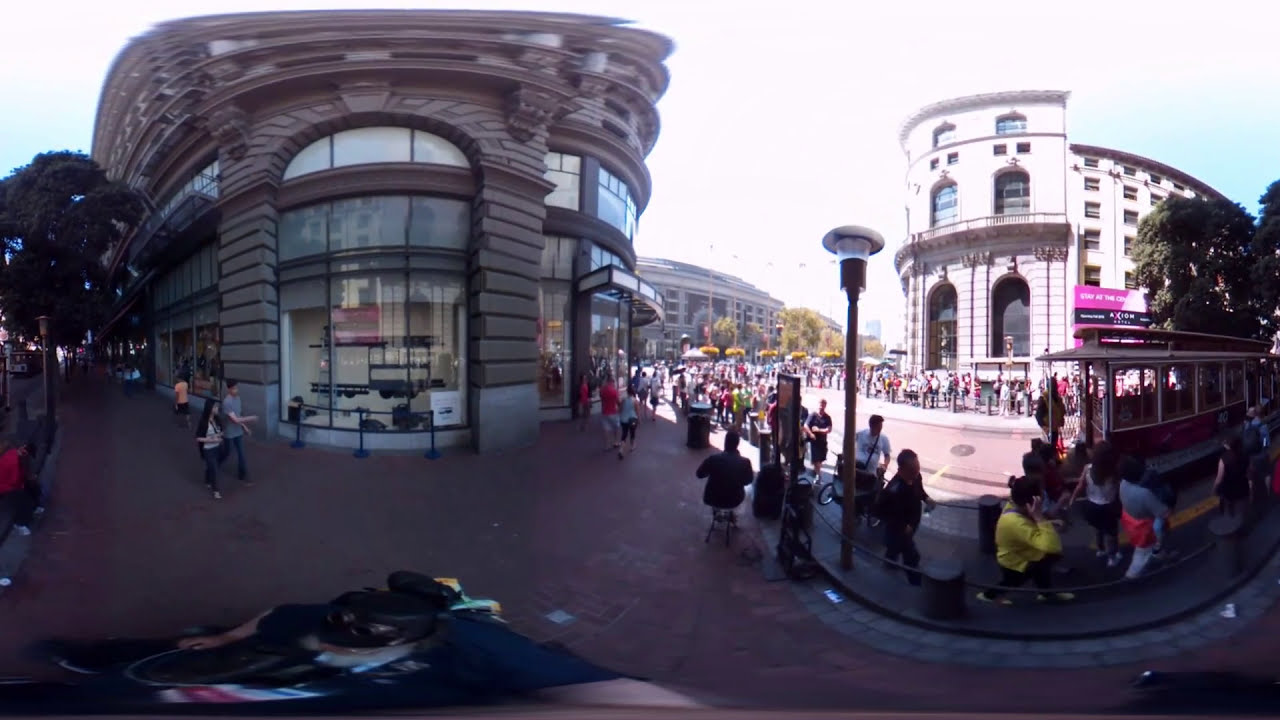This panoramic photograph captures a bustling city street with distinct European architecture. To the left, there is a tan brick building with large, see-through windows that resemble store displays, featuring blue chain-linked posts outside. In front of this building, a person wearing a blue shirt and pink and white skirt or shorts sits on the sidewalk, while other pedestrians, dressed in various colors including gray, black, peach, and red, walk by. A prominent tree with green foliage and a brown stem stands at the far left.

In the background, merging to the right, stands a classical-style building with stone and brick columns and archways, adorned with large glass windows. The building on the right is brightly lit by the sun, appearing almost white, while its windows and doors contrast with darker hues. The sky above shifts from a light turquoise blue at the edges to a bright white near the center due to the intense sunlight.

Further down the street, a vivid red and cream old-style single-decker tram with wide windows can be seen. Scattered throughout the scene are numerous people, some wearing yellow, blue, red, white, and black shirts, emphasizing the busy, energetic atmosphere of the city. The distant background showcases several large, stone buildings that complement the architectural theme of the scene. An unreadable sign with black, red, and white writing adds to the urban setting. The overall image captures a vibrant snapshot of everyday life in a picturesque city environment.